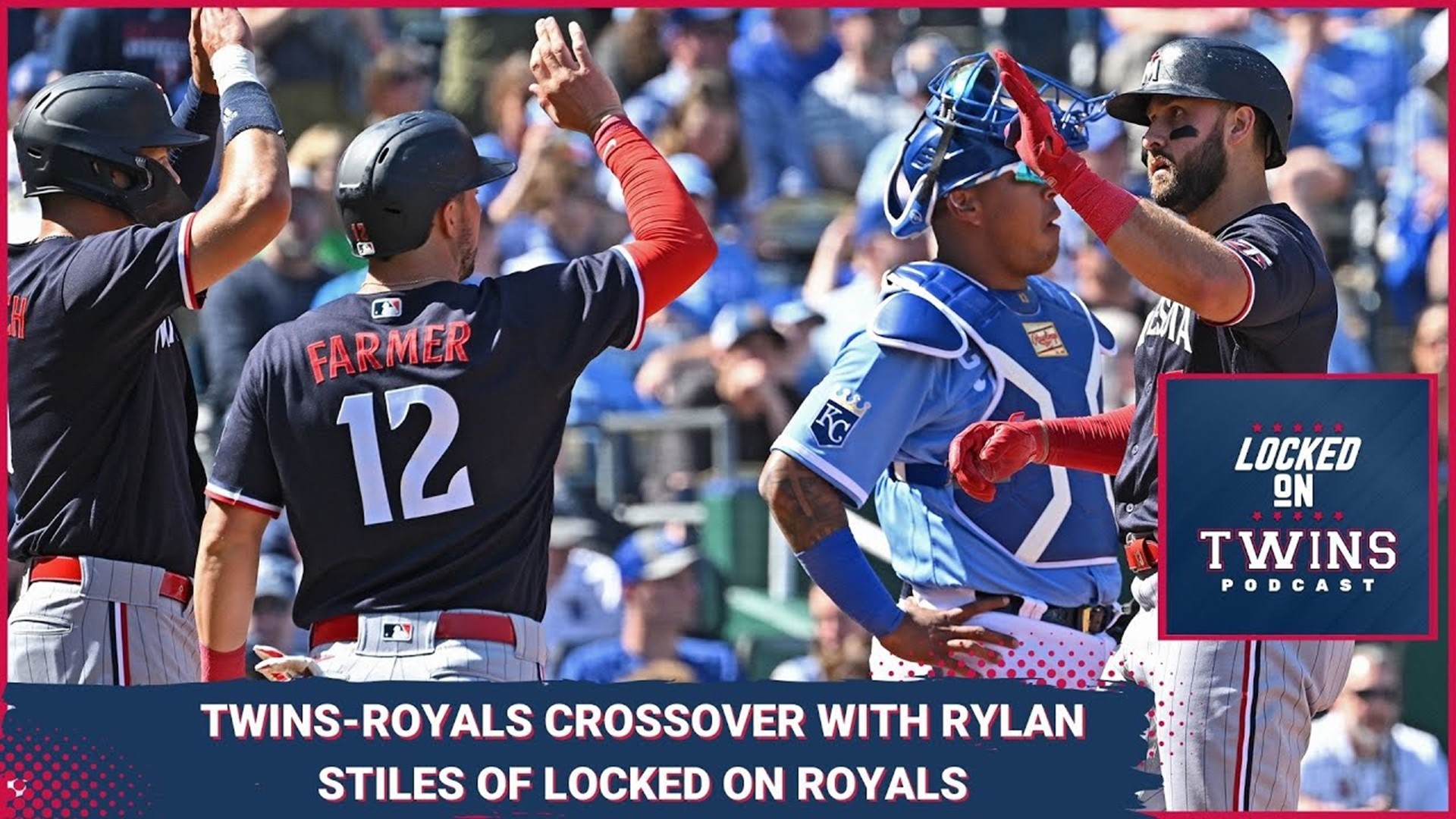The image captures a lively moment at a baseball game featuring three players in black helmets and navy jerseys with gray striped pants, accented with red, white, and blue trim around the cuffs. The player in the center has his back to the camera, displaying "Farmer" and the number 12 in red on his jersey, while the MLB logo is visible on the back of his pants. All three players are raising one hand for high-fives. To the right, a player in a blue jersey and helmet, bearing the Kansas City logo, stands beside them. An umpire, dressed in a white shirt and pants, stands with his hands on his hips in the background. Behind them, the spectator area is packed with fans predominantly dressed in blue. At the bottom of the image, text reads, "Twins Royals Crossover with Ryland Styles of Locked On Royals," and on the right side, a blue square states, "Locked On Twins Podcast."